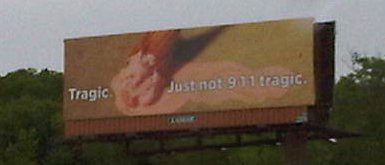The image depicts a horizontally cropped, lower resolution photograph of an outdoor advertisement banner, displayed on a billboard along a roadside or highway. The scene is set against a backdrop of gray skies and green trees, adding a somewhat melancholic atmosphere. The billboard features a pastel-colored image of a fallen strawberry ice cream cone, melting onto a brownish-yellow surface. The ice cream, with a visible waffle cone, appears tragically abandoned. Above the melting cone, white, bubbly text reads: "Tragic," followed by, "just not 9-1-1 tragic" to the right of the image. The billboard is positioned on a metal base attached to a backboard with vertically striated lines, underlined by a brown section. Overall, the image conveys a message about overreacting to minor misfortunes with a mix of visual irony and mild humor.